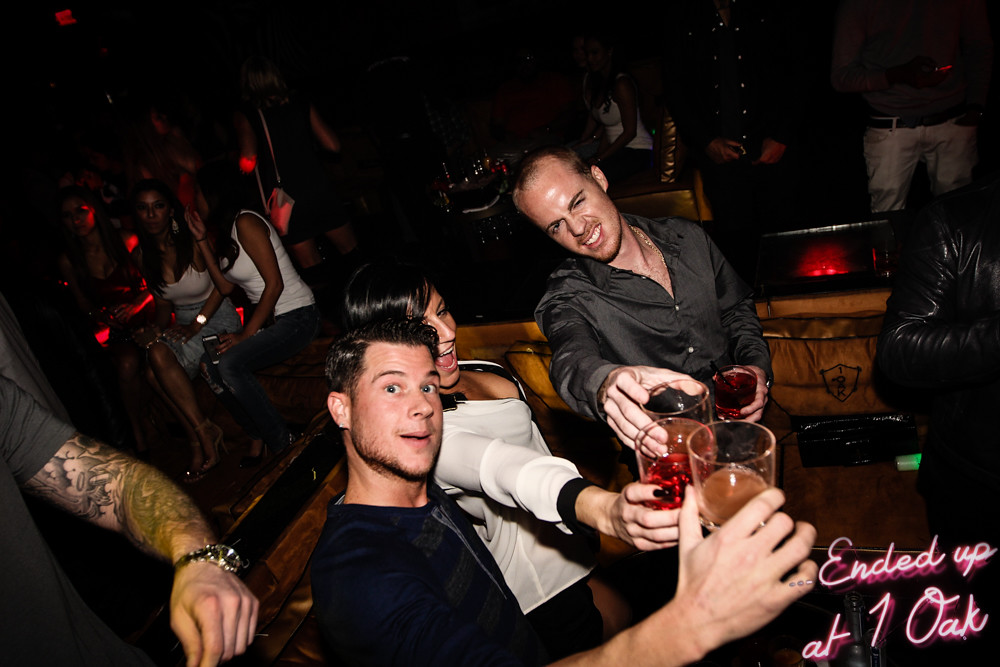In a dimly-lit nightclub, three people are seated at a table within a booth, centered in the image, toasting with shot glasses in a lively, casual manner. On the far left, a man's tattooed arm wearing a watch is visible. The man closest to the camera sports spiky hair and a black shirt, raising his glass toward the lens. Behind him, a woman in a white v-neck top is smiling and holding up her drink. She is flanked by another man in an unbuttoned gray button-up shirt, showcasing a gold chain and a balding head, who is holding up two drinks with a sneer. In the blurry background to the left, clusters of people including some girls in white tank tops can be seen. Additional figures in white and khaki are also faintly discernible. The bottom right corner of the photo features neon-accented text, "ended up at one oak," highlighting the spontaneous and joyful nature of the scene.